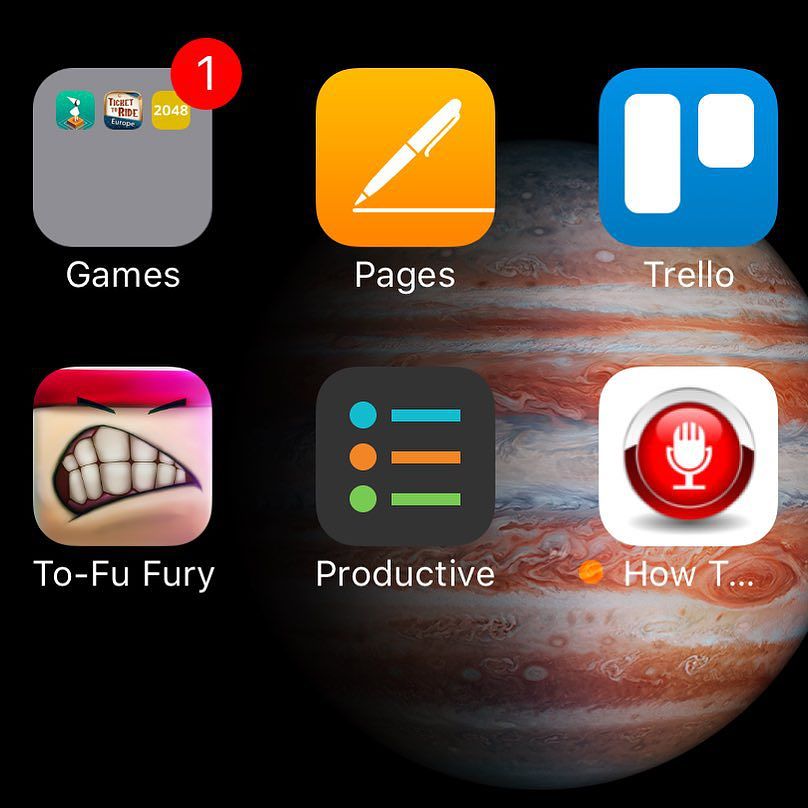The image appears to be the home screen of a digital device such as a smartphone or computer. The background is a solid black, accentuating a visually striking planet in the center. The planet features a mix of gray and red hues, with intricate details such as bubbles, assorted shapes, twists, and tornado-like formations, with subtle hints of blue throughout.

App icons are strategically placed along the lower section of the screen. Starting from the left, there's a gray square labeled "Games" in white text, featuring three distinct icons and a red notification circle with a white "1" inside. Next is a brown square labeled "Pages," adorned with a white ink pen drawing. To the right, a blue square labeled "Trello" displays two vertical white lines.

Adjacent to it is a pink square with a humorous graphic resembling a character having a pink headband, two black eyebrows, and a large mouth with prominent teeth, labeled "Tofu Fury." Following that, there is a black square with intersecting blue, orange, and green lines ending in dots, labeled "Productive." Finally, a white square with a red circle containing a microphone icon is labeled "How To."